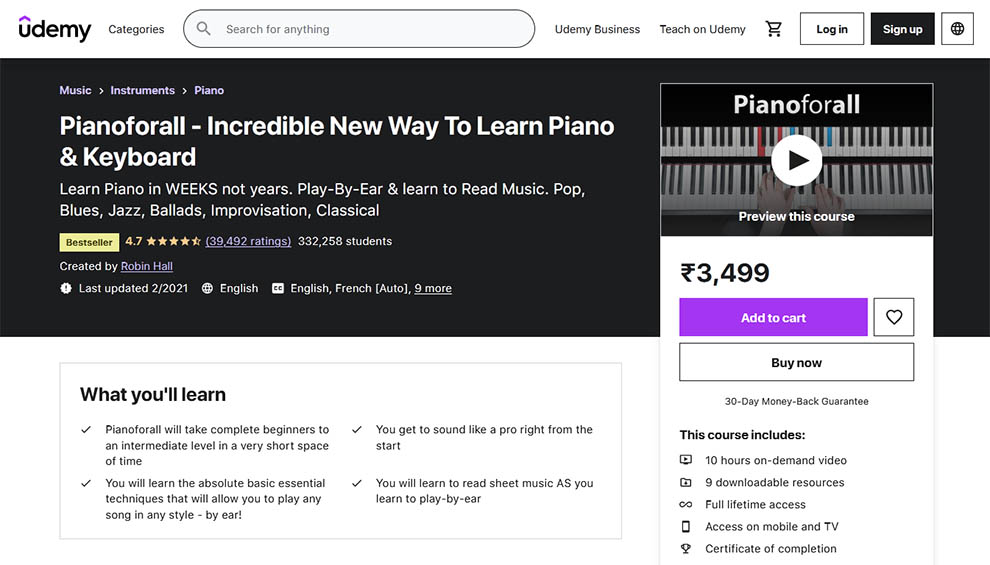This image is a screenshot from the Udemy website, found at "Udemy.com". The header features various elements including category links, a search bar, options for Udemy Business, and a "Teach on Udemy" section. Additionally, there is a shopping cart icon and buttons to log in or sign up, situated towards the right of the header. 

Dominating the central part of the webpage is a black rectangular banner promoting a piano course. The banner's text highlights "Music", "Instruments", and "Piano", specifically focusing on a course titled "Piano For All: Incredible New Way to Learn Piano and Keyboard". The course promises students they can "Learn Piano in WEEKS, not years", emphasizing the word "WEEKS" in all capital letters. It also mentions that students will learn to play by ear, read music, and explore genres such as pop, blues, jazz, ballads, improvisation, and classical music.

Below this description, there is a video labeled "Piano For All" with a prompt to "Review this course". The price for the course is stated as "₹3,499" (denoted by a squiggly line with two stripes through it), with an "Add to Cart" button in purple, and a "Buy Now" option available. A heart icon, presumably for adding the course to a wishlist, is also displayed.

Further down, there are sections detailing "This course includes" and "What you'll learn", although the specific content of these sections is not fully visible in the screenshot.